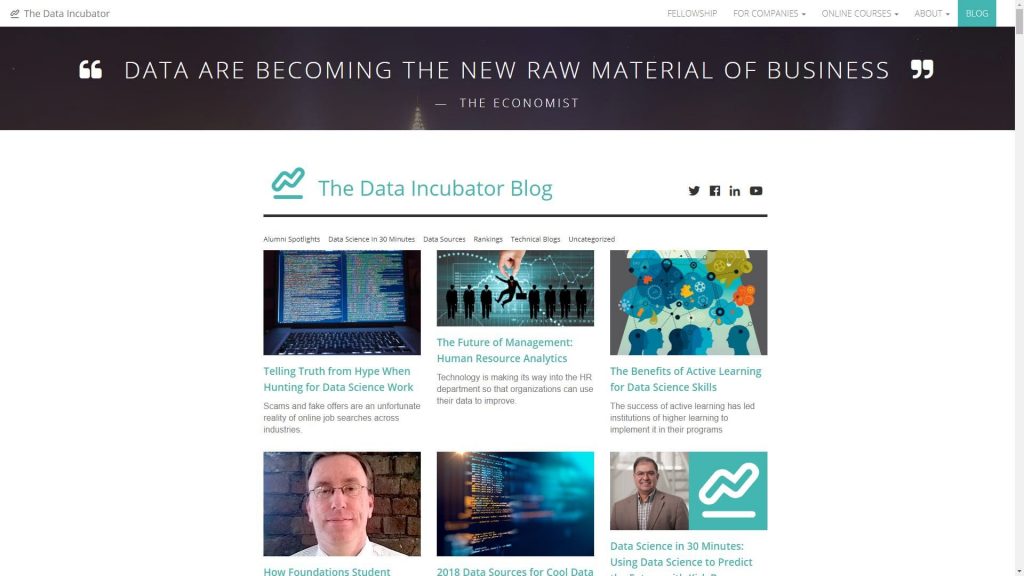This image is a color, landscape-format screenshot from a computer displaying the website of "The Data Incubator." The text "The Data Incubator" is prominently featured in black lettering, accompanied by a modest logo on the left, designed with a simple zigzag pattern. At the top, a notable quote from The Economist reads, "Data are becoming the new raw material of business."

The website navigation bar includes tabs for "Fellowship," "For Companies," "Online Courses," "About," and "Blog." Below this, the section titled "The Data Incubator Blog" showcases a series of featured articles. Six articles are visible, each accompanied by generic tech-related images. The article headlines visible in the screenshot are:

1. "Telling Truth from Hype and Hunting for Data Science Work"
2. "The Future of Management: Human Resource Analytics"
3. "The Benefits of Active Learning for Data Science Skills"
4. "How Foundations Student..."

The remainder of the articles would require scrolling further down the webpage to view.